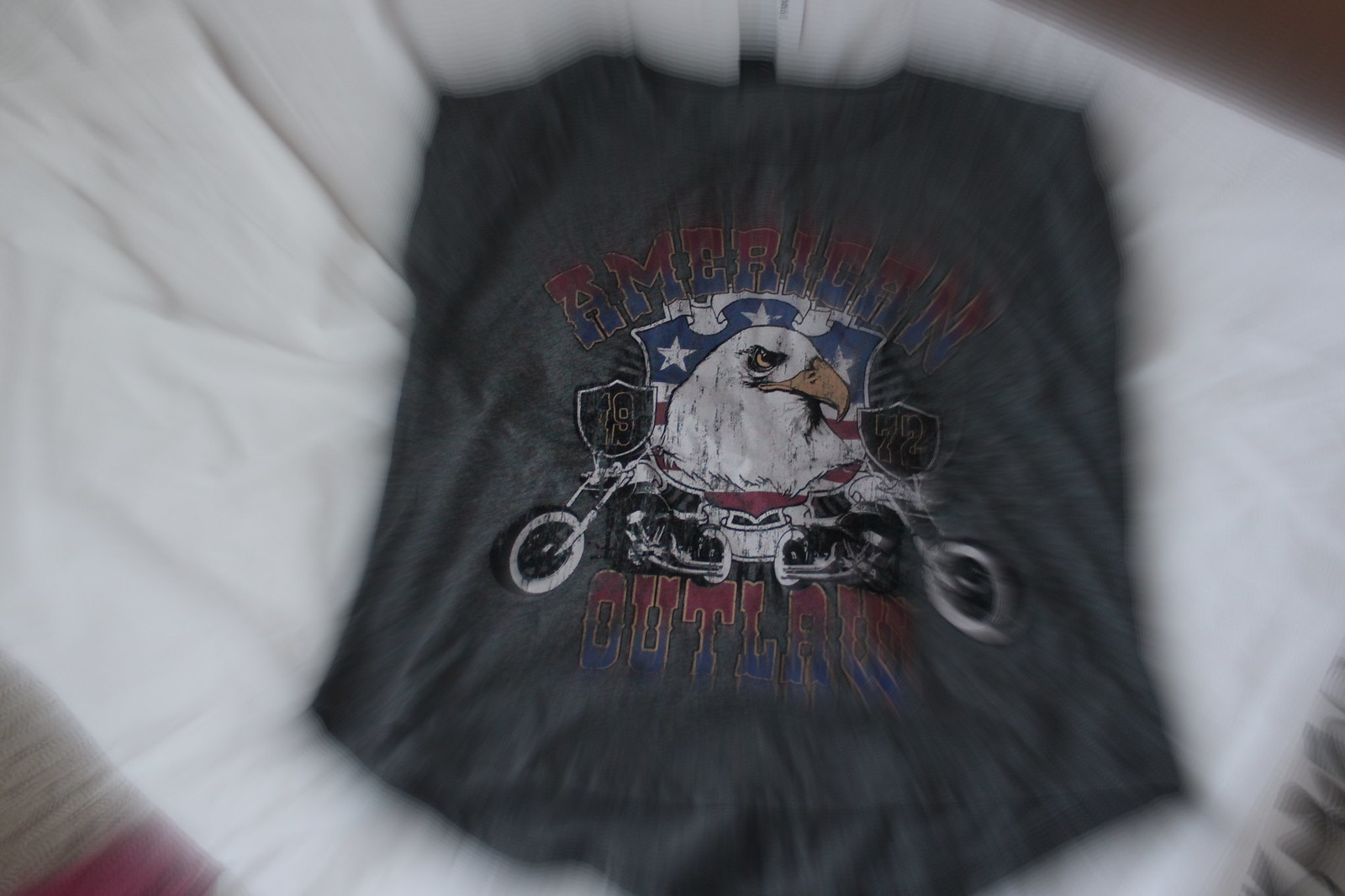This photo depicts a folded gray t-shirt placed on a white, possibly blurry background. The central design on the shirt features a white eagle draped with an American flag. Surrounding the eagle are two black shields displaying the numbers 19 and 72. Beneath these shields, there are images of two motorcycles, likely resembling Harley Davidsons, positioned on the left and right side of the design. The text "American Outlaw" is prominently displayed in a gradient of red to blue, with "American" at the top and "Outlaw" at the bottom. Additionally, stars can be seen behind the eagle, enhancing the patriotic theme.